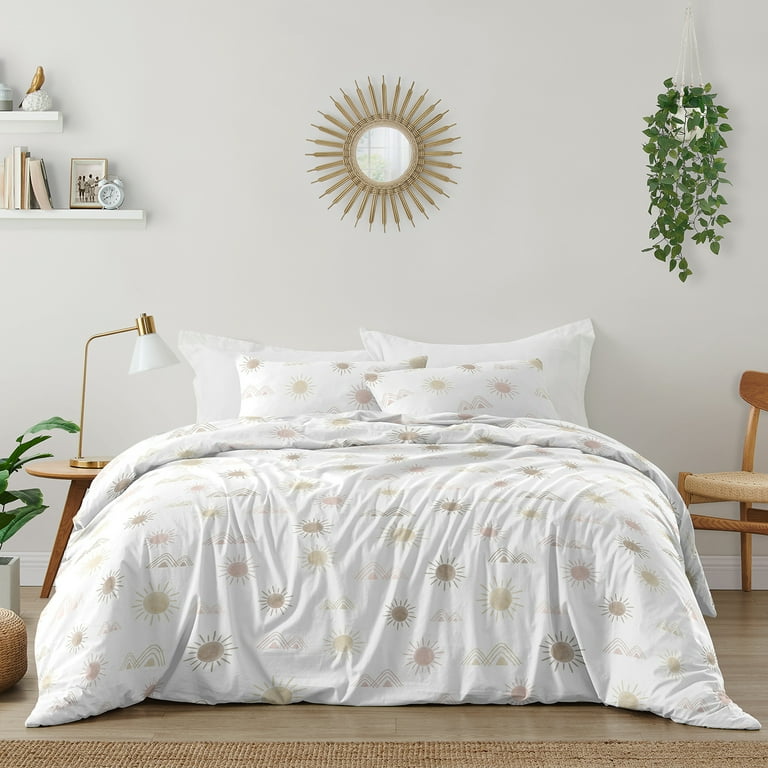This color photograph showcases a serene bedroom centered around a spacious bed, draped in a white bedspread adorned with gold-inked prints of suns and mountains. Four pillows rest at the head of the bed, which, notably, lacks a headboard or footboard. Positioned on the left side of the bed, a small wooden side table holds a white and brass lamp. Above the bed, a striking golden sunburst mirror graces the white wall. To the upper right, vibrant ivy plants hang elegantly from the ceiling, and below them sits a wooden chair on the natural jute rug that covers the wooden floor. On the wall to the upper left, two white bookshelves display various tchotchkes and books, adding a personal touch to the minimalist decor.